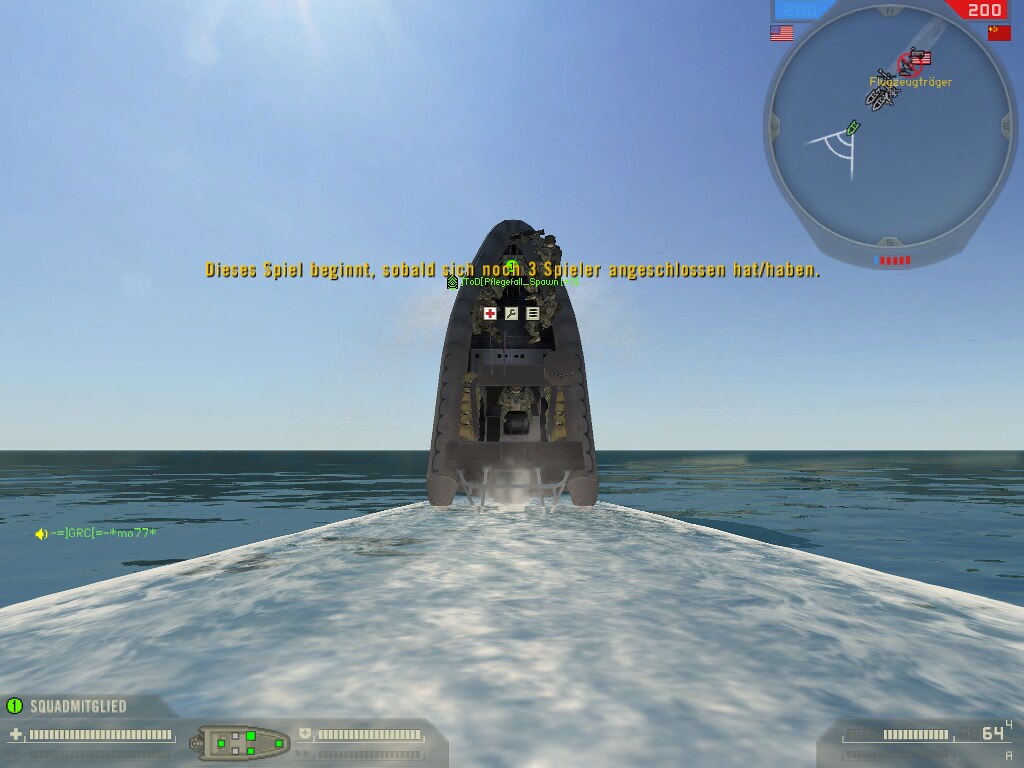In this action-packed video game screenshot, the scene captures an intense moment out on the open ocean. The focal point of the image is a speeding boat at the center, so fast that it appears almost vertical, with its nose pointing skyward and the boat's interior visible. The sky is a bright, clear blue, illuminated by a light source shining down from the top-left corner. 

In the bottom-right corner of the screen, a game interface displays a health bar indicating "64." Nearby, a red indicator bar annotated with "200" in white print stands out. The top-right corner features a circular map showing the player's green boat heading towards the bottom-left corner, accompanied by what looks like sonar pings. Positioned behind the player's boat on the map is another vessel, alongside a distinct red circle crossed out by a line, indicating a potential threat or no-go area.

In the bottom-left corner, the word "squad" is displayed beside "MITGLIED," suggesting a team or multiplayer element. This is paired with a simple boat icon facing right, marked with small green rectangles likely representing teammates or status indicators. Every detail of this image showcases a dynamic and immersive gaming experience, filled with action, navigation, and strategic elements.